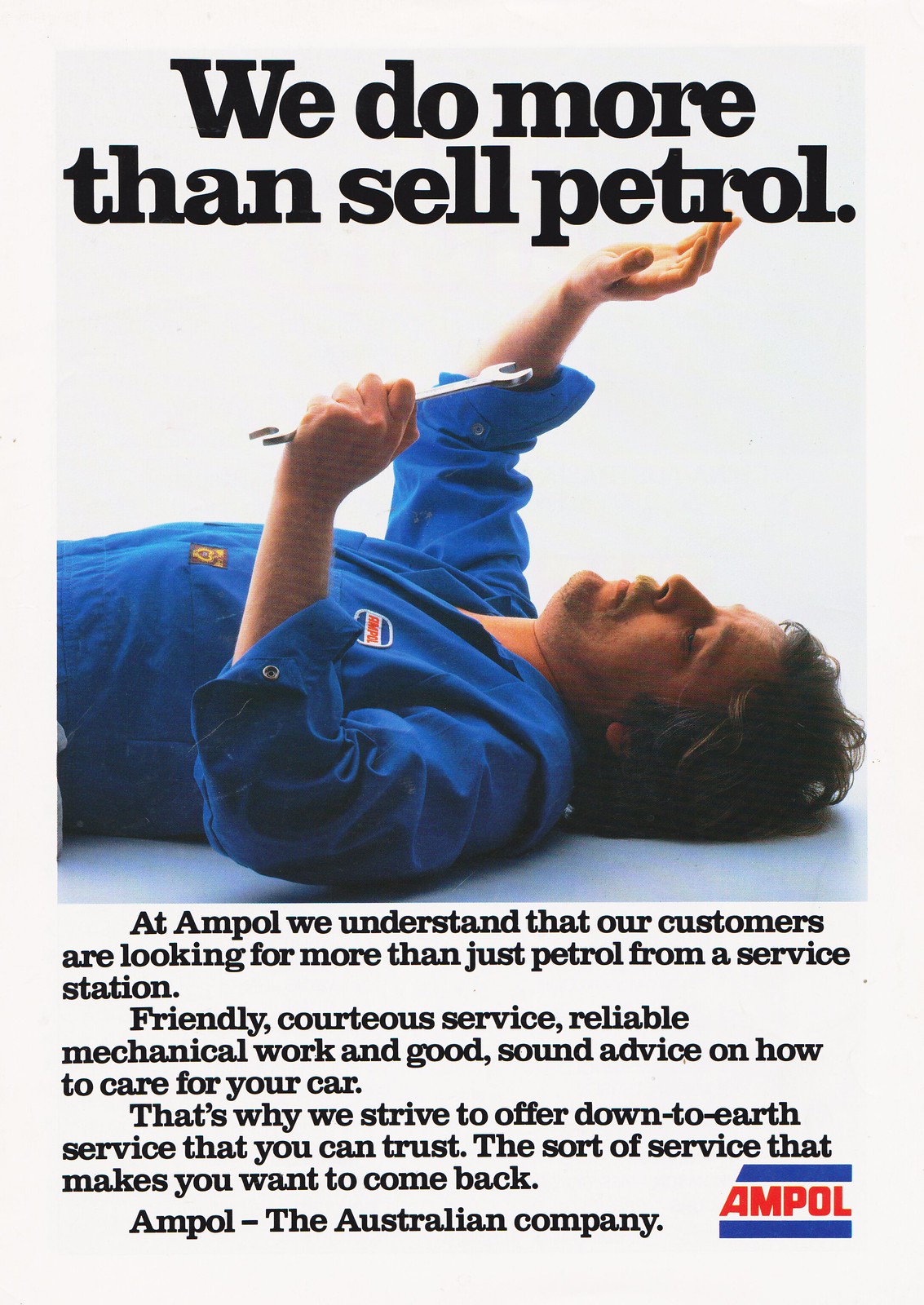This vertical, rectangular advertisement for Ampol prominently features the company's logo in the bottom right corner. The logo consists of bold red letters spelling "Ampol," flanked by thick blue lines above and below, with a diagonal slant at one end. The central photograph captures a man in blue coveralls, identifiable as a mechanic, lying on his back as if working underneath a car, though the car is not visible. He has brown hair, a mustache, and is holding a wrench in his left hand, appearing to inspect something. Above him, in large black letters, the tagline reads, "We do more than sell petrol." Below the image, additional black text explains Ampol's understanding that customers seek more than just petrol from a service station, emphasizing their dedication to providing friendly, reliable service and sound car maintenance advice. The text reiterates that Ampol is "the Australian company," reinforcing their commitment to trustworthy and down-to-earth service.